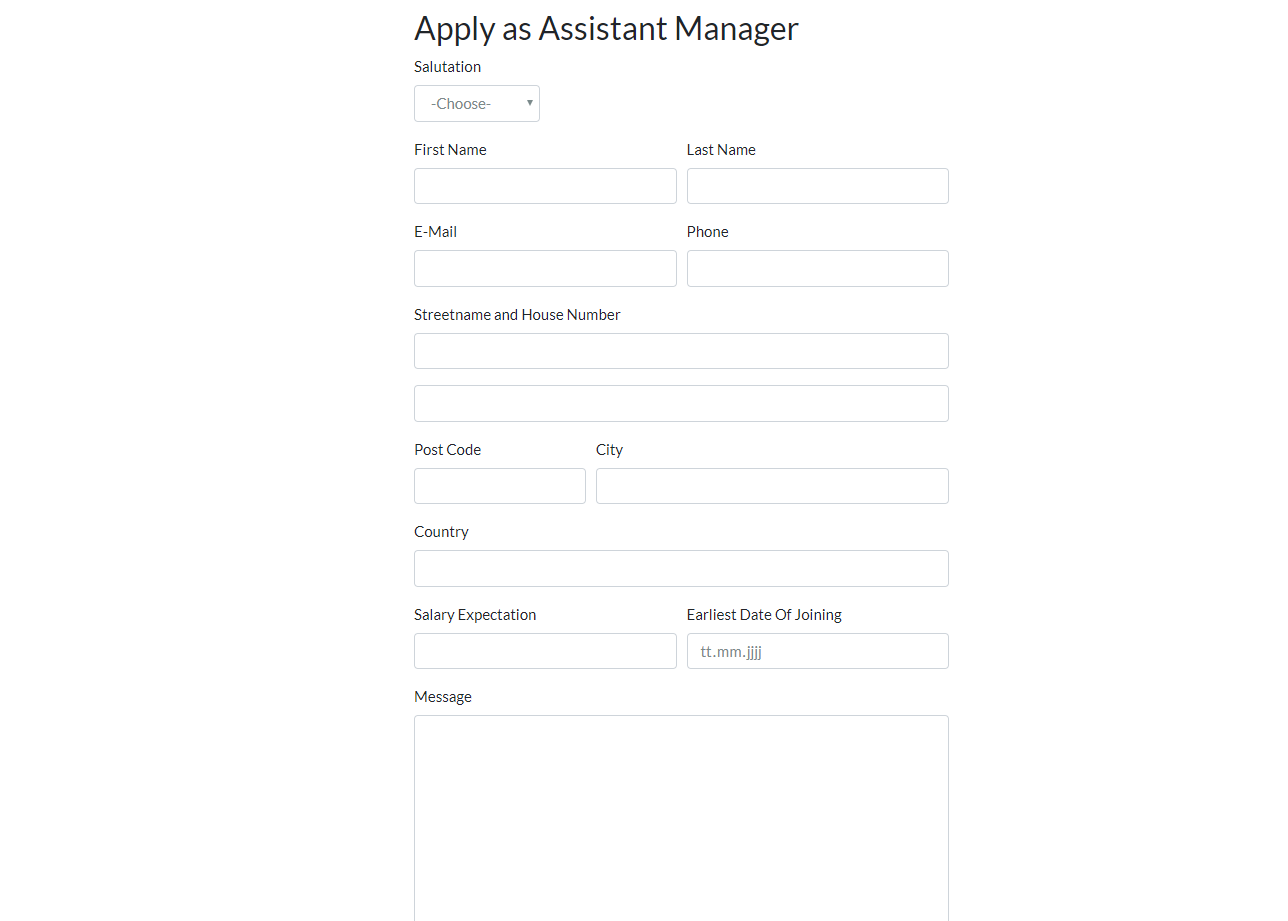### Descriptive Caption:
The image features a vertically oriented, predominantly white form with black text designed for applying to an Assistant Manager position. At the top, bold black letters emphatically display the instruction "Apply as Assistant Manager." 

Below this heading, aligned to the left, the word "Salutation" appears in black, accompanied by a drop-down menu labeled with gray text that reads "Choose." This menu allows applicants to select their preferred salutation. 

Following this, the form fields for personal details are arranged methodically. The "First Name" field, placed to the left, features a text box for input. Adjacent to it on the right is the "Last Name" field with another text box. Directly below the "First Name" field, the "Email" field appears with its corresponding text box for input, and to its right is the "Phone" text box.

Further down, there are two text boxes for entering the "Street Name and House Number." Below the second text box, "Post Code" is listed on the left with its text box beneath it, while to the right, "City" is labeled with an elongated text box for detailed entry. 

Continuing sequentially, directly underneath the "Post Code" field is the "Country" field, featuring another extended text box. 

The form proceeds to prompt for "Salary Expectation" with a text box below this label. To the right of the "Salary Expectation" field, "Earliest Day of Joining" is indicated in black letters. This section includes a date input field represented by placeholders typically shown as "TTMMJJ" in gray letters.

Finally, at the bottom of the form is a "Message" section indicated by black letters, inviting applicants to type into a large text box that partially extends out of the image's visible area.